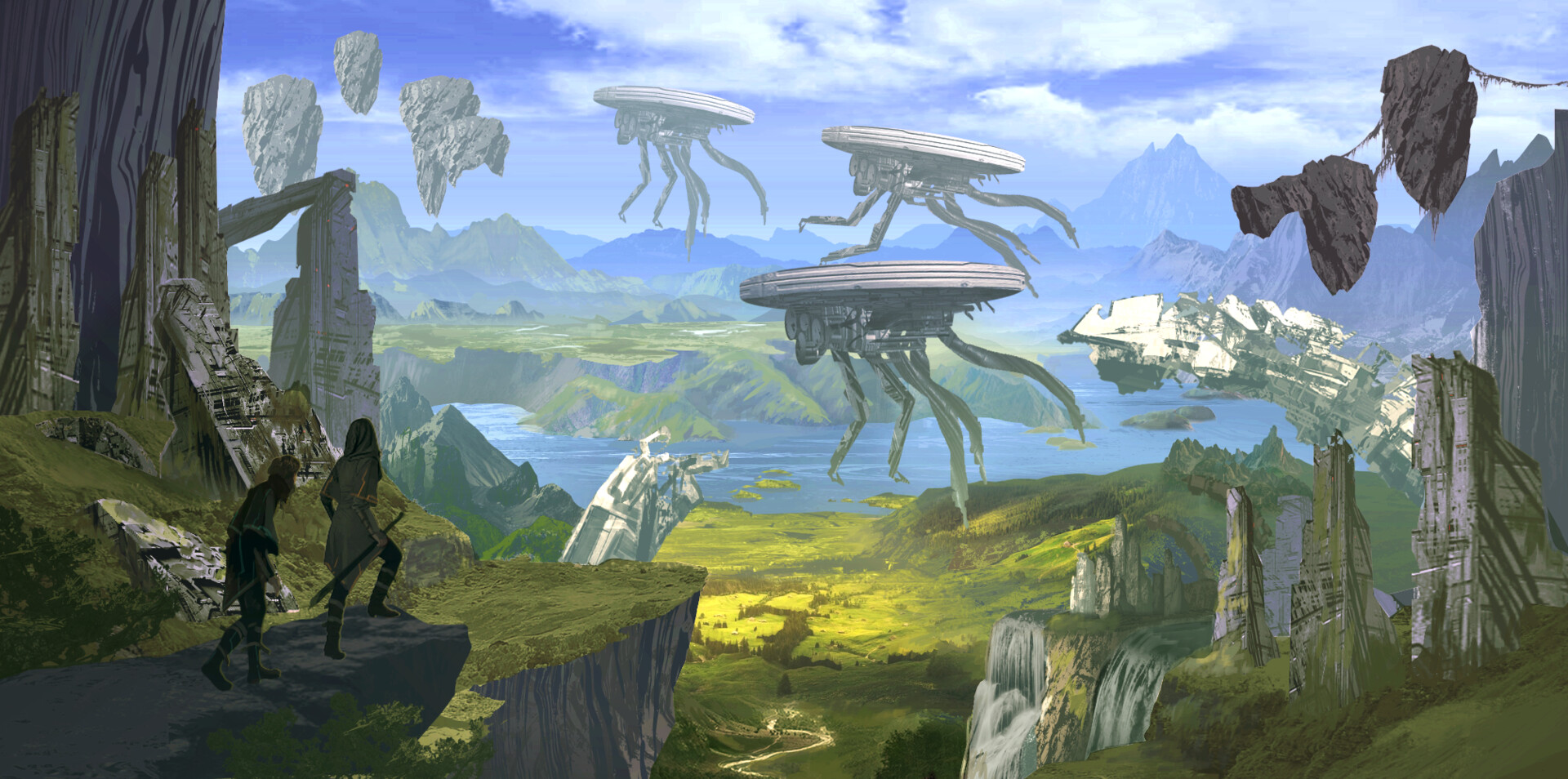The artwork is a detailed, surrealistic outdoor scene that blends elements of science fiction and dystopian fantasy. Dominating the left-hand side is a massive tree trunk and a rocky plateau where two human figures, clad in medieval garb from the 1400s or 1500s, stand gazing at the sky. The scene includes jagged, spiked rock formations jutting up from the ground on the right side, set against a blue and green sky. Floating in the air are three mechanized creatures resembling a hybrid of insects and steel platforms, each with multiple legs and descending tentacle-like appendages. The creatures appear to be moving from the bottom right to the top left, catching the attention of the two figures below. The landscape also features a grassy mesa overlooking a lush, green valley with a winding river and floating mountain structures, hinting at a dystopian world with remnants of destroyed buildings. The background reveals more rocky outcroppings and mountains, completing the fantastical, otherworldly tableau.